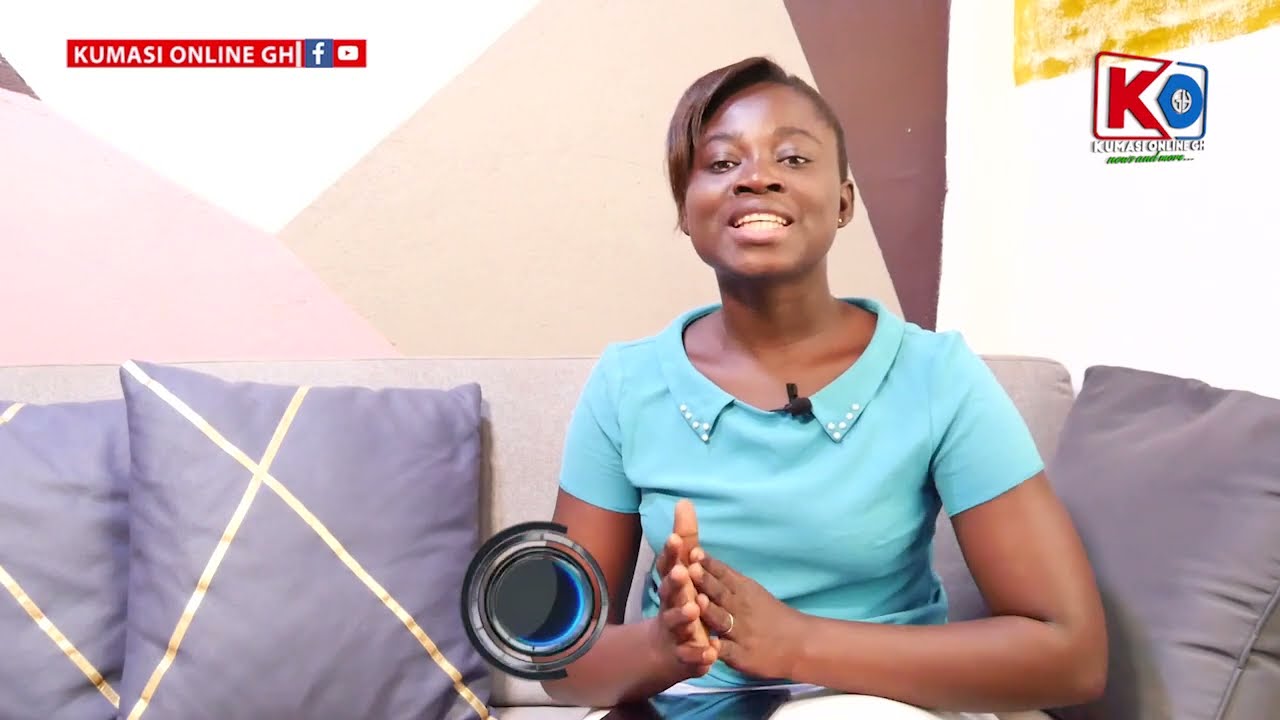The image depicts a young woman with short, dark hair and a darker skin complexion, seated on a gray couch adorned with bluish-gray pillows on her right and light blue pillows with white X's on her left. She is wearing a light blue short-sleeved shirt with a collar and a small microphone pinned to it, indicating that she is engaged in a conversation. Her hands are together, revealing a ring on her left ring finger. She appears to be looking at the camera while speaking.

The background features an abstract pattern with colors ranging from brown to beige, light pink, and white. The top right corner includes a logo with the letters "KO" in red and blue, and the words "Kumasi Online" underneath. The top left corner displays text that reads "Kumasi Online GH," accompanied by Facebook and YouTube icons, along with additional red and white outline letters. There is also a black circle with some blue near her arm, which could either be on the screen or in front of her.